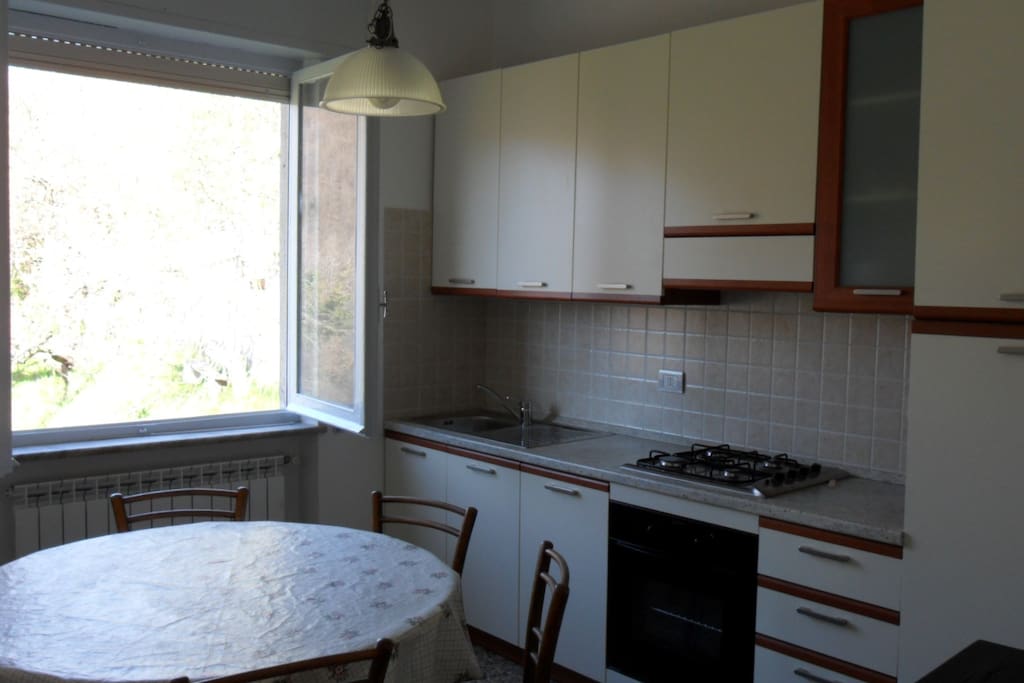The photograph showcases a somewhat dated kitchen with a distinct 90s aesthetic. The main focus is a round table in the lower left corner, covered with a white vinyl or plastic tablecloth, surrounded by four wooden chairs. An open, inward-hinged, white window behind the table allows bright sunlight to flood the room, with visible trees and branches outside. A dome-shaped light fixture hangs from the ceiling above the table, though its bulb appears to be out.

The overall palette of the kitchen consists of white and brown. The cabinets, which feature brown wood trim, are positioned above the silver sink and next to a stove top with a black and white oven beneath it. The backsplash behind the sink and stove adds to the dated look with its darker cream tile. A plug outlet is situated to the right of the sink and to the left of the stovetop, contributing to the practical, though somewhat aged, functionality of this kitchen.